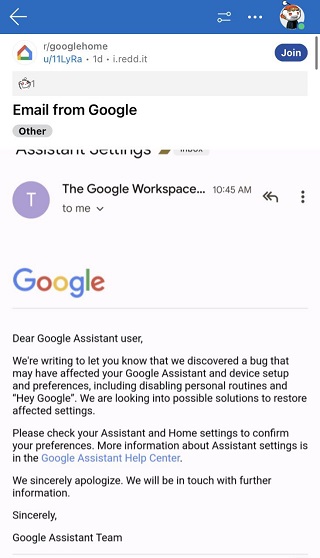Phone Screenshot of Google Home Email Notification

In this screenshot captured from a smartphone, there is an email notification displayed prominently. Starting at the top, a blue navigation bar features a left-pointing arrow and a small, circular icon resembling a child-like robot situated on the far right.

Below the navigation bar, in bold black lettering, the subject line reads "r/Google Home" followed by "Email from Google". This is highlighted in a gray box labeled "Other." Next, a purple box indicates "Google Workspace," with the recipient marked as "to me."

The body of the email, against a white background, prominently features the word "Google" written in its characteristic multi-color logo. The message then begins with a formal greeting, "Dear Google Assistant user," and proceeds to inform the user of a discovered bug. The bug potentially affected the user's Google Assistant and device setup, including disabling personal routines and the "Hey Google" feature.

The email explains that Google is working on solutions to restore the affected settings and advises users to check their Assistant and home settings to confirm their preferences. It also directs users to the Google Assistant Help Center for more details. The message concludes with an apology and a promise of further communication, signed by "Sincerely, the Google Assistant team."

The overall background of the email remains white, ensuring a clean and straightforward presentation of the information.